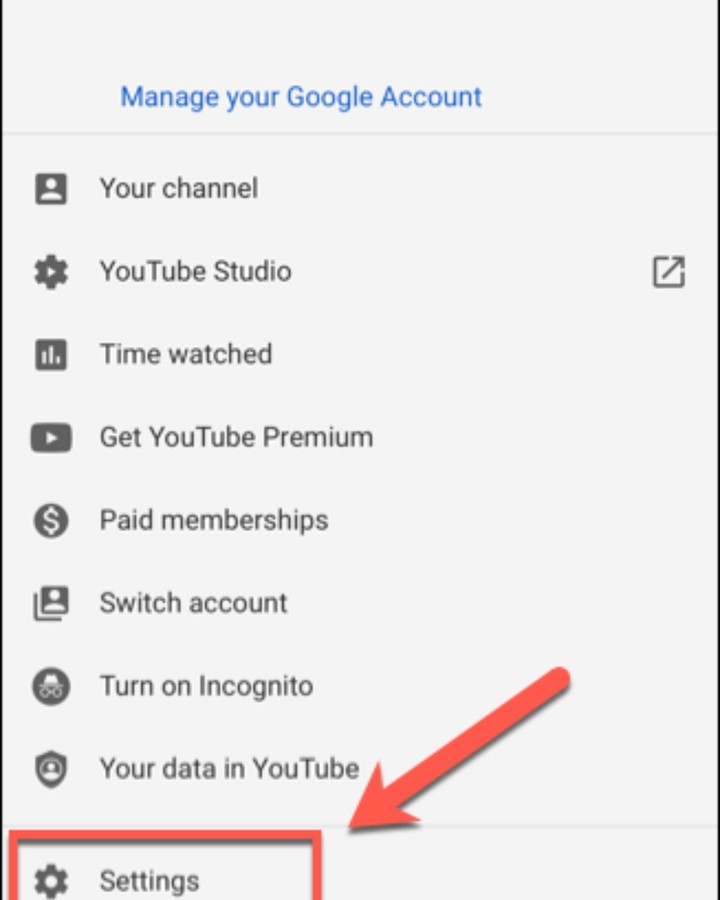The image is an instructional screenshot designed to guide users on how to navigate to the settings on their YouTube account. The screenshot features an off-white background and presents only a partial view of the interface. At the very top of the image, in blueprint text, the label "Manage your Google Account" is prominently displayed. 

Below this header, a vertical list of icons with accompanying text is visible. Each icon is rendered in gray and white. From the top to bottom, the icons and their labels are as follows:

1. A stick figure man icon labeled "Your Channel."
2. A cogwheel with a small play icon labeled "YouTube Studio."
3. A bar graph icon labeled "Time Watched."
4. The YouTube play icon labeled "Get YouTube Premium."
5. A circular icon with a dollar sign labeled "Paid Memberships."
6. A square icon featuring a person, similar to the "Your Channel" icon, labeled "Switch Account."
7. An icon of a person wearing a private investigator hat and glasses labeled "Turn on Incognito."
8. An avatar icon inside a shield labeled "Your Data in YouTube."
9. A final cogwheel icon labeled "Settings," which is highlighted with a red square and pointed at by a red arrow.

Additionally, the right side of the menu includes a pop-up extension option to reveal more items. The primary focus of the screenshot is the "Settings" option, denoted by the red highlights, guiding users specifically to this menu item among various YouTube settings and choices.